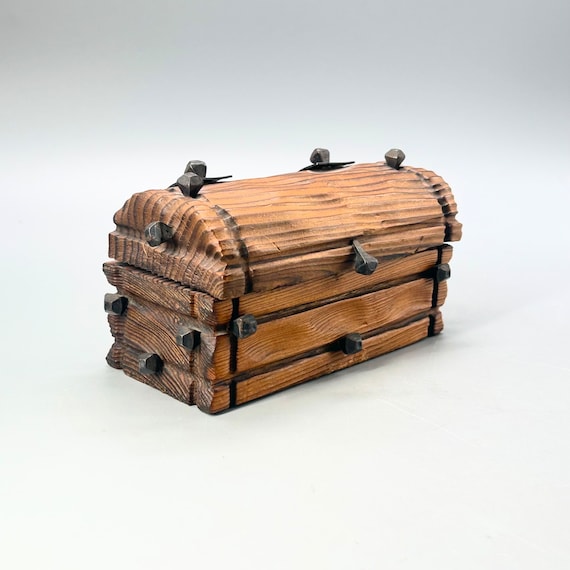In this professionally taken photograph, a wooden treasure chest is prominently displayed against a background that transitions from a medium gray at the top to a very light gray at the bottom. The chest is positioned diagonally, revealing both the front and one of its sides. It features horizontal slats of medium brown wood with darker wood strips creating borders between each slat. The top of the chest is slightly rounded and appears to be textured and grooved, showcasing natural wood grains. The chest is accented with numerous black metal pieces, possibly screws or bolts, that add a contrasting detail to the rustic wood. The lighting and resolution of the image highlight the natural patterns and slightly rough edges of the chest, suggesting it is an authentic, possibly antique, item.